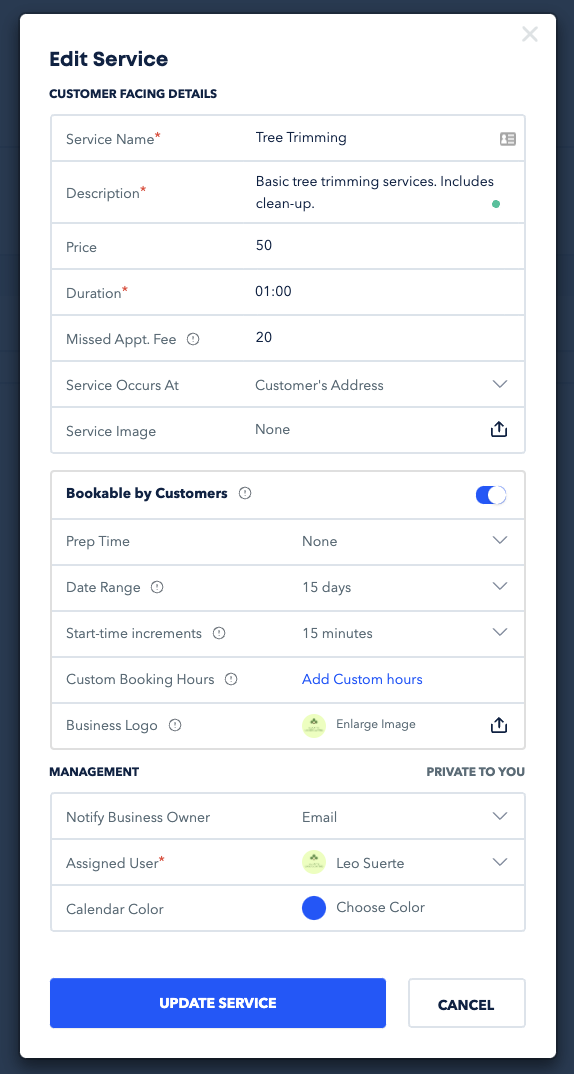The image depicts an options page within a mobile app designed for a tree trimming service, featuring a variety of editable fields and settings for service customization and customer booking:

1. **Edit Service**:
   - **Service Name**: A mandatory field marked with a red asterisk, filled in with "Tree Trimming."
   - **Description**: Also mandatory, stating "Basic tree trimming services includes cleanup."
   - **Price**: Listed as "50" without a currency symbol, presumably USD.
   - **Duration**: Another mandatory field, marked with an asterisk, set to "01:00" for one hour.
   - **Missed Appointment**: Labeled as "APPTV" with a clickable question mark icon for more information, set to "20."

2. **Service Occurs At**:
   - Specified as the "Customer's Address" with a dropdown caret icon for additional details.

3. **Service Image**:
   - Indicated as "None" with an upload icon on the far right for adding an image.

4. **Bookable by Customers**:
   - Marked with a question mark icon for more details and featuring a white and blue toggle switch for enabling or disabling customer booking.

5. **Additional Fields**:
   - **Prep Time**: Listed as "None."
   - **Date Range**: Set to "15 days."
   - **Start Time Increments**: Set in 15-minute intervals.
   - **Custom Booking Hours**: Option to "Add Custom Hours" highlighted in blue font.
   - **Business Logo**: Displaying the company's logo with an option to upload a new image.

6. **Management**:
   - **Private to Use**: For internal use by the vendor.
   - **Notify Business Owner**: Options available presumably via email, adjustable with a menu icon.
   - **Assigned User**: Featuring a small company logo and the name "Leo Suerte."
   - **Calendar Color**: A dark blue color selectable for calendar events.

7. **Action Buttons**:
   - Blue "Update Service" button and a "Cancel" button to the right.

This highly detailed options page allows for comprehensive customization of tree trimming services, ensuring both business and customer needs are met efficiently.